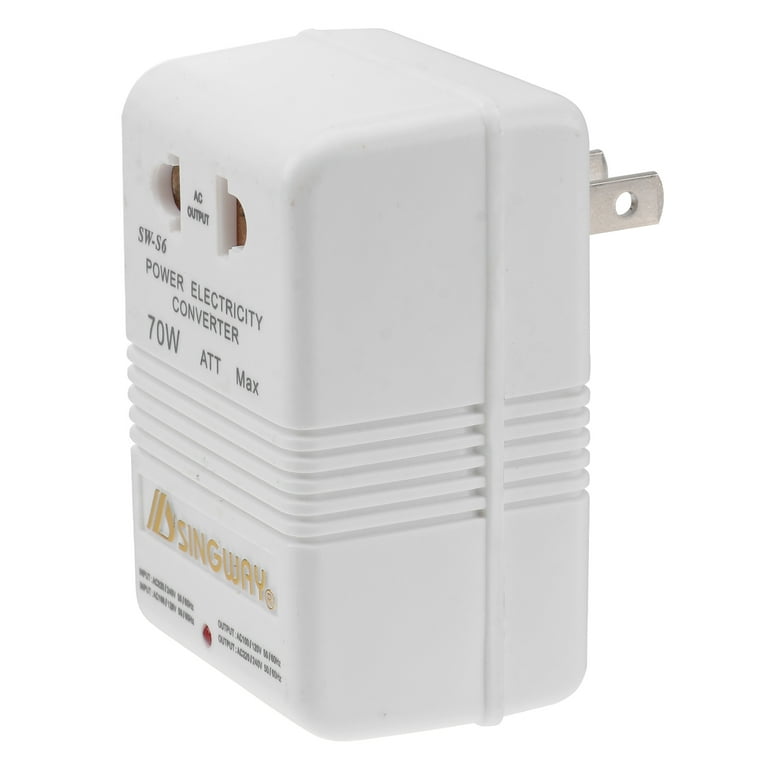The image depicts a white Singway power electric converter, specifically model SW-S6, designed to convert American to British power. The converter has two American prongs on the back and a European British female connector on the front, labeled "AC output." Beneath this, there is the text "70 watts ATT max." The device also features the Singway logo in yellow at the bottom, which includes a red indicator light to show whether the converter is plugged in and operational. The overall color is a faded white-gray, with six grip lines on the sides to assist in plugging the converter in. The image captures the detailed textures and depth of the physical device, making the text and design elements, like vents and warning signs, visible but not entirely readable.